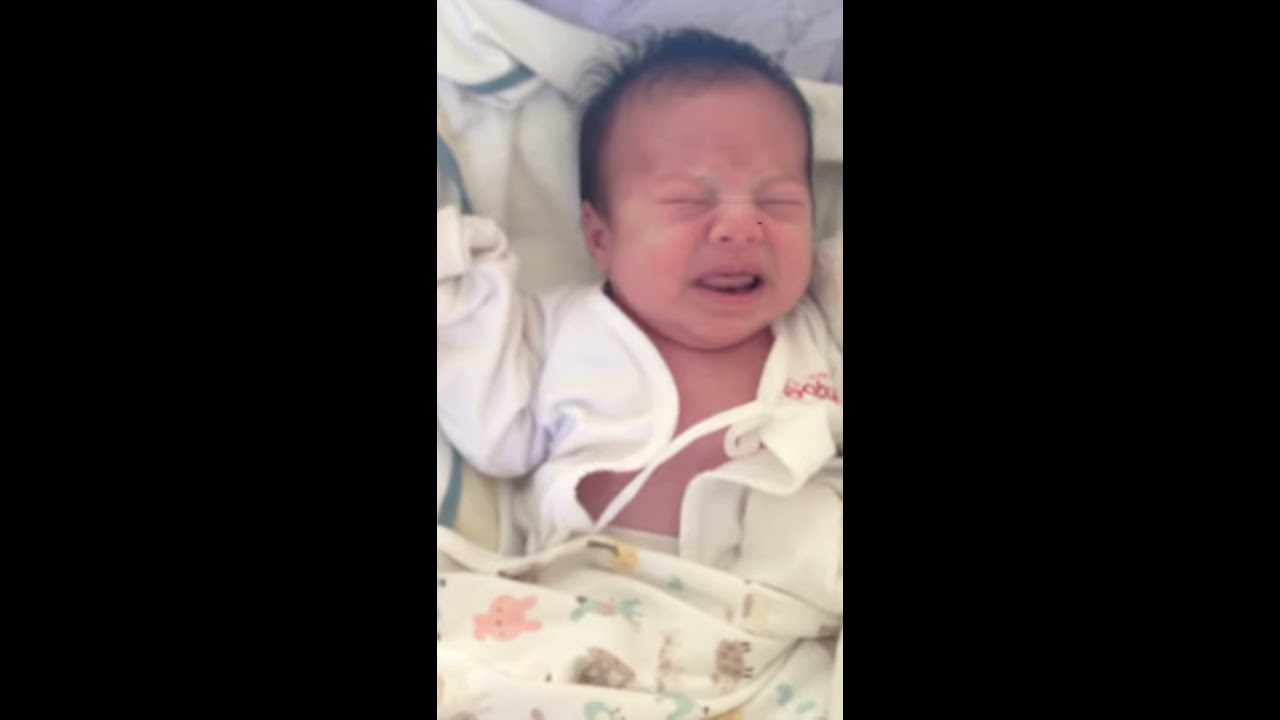This image features a newborn baby laying on its back, dressed in a white robe that seems too large, enveloping their tiny frame. The robe opens at the center, revealing the baby’s very pink skin, while the long sleeves partially obscure their hands. The infant, with thin dark hair, appears to be crying; their eyes are squeezed shut and their mouth is open, with the tongue peeking out slightly. The baby's face is scrunched up from crying.

The newborn is nestled among several blankets. A white blanket, adorned with small animal illustrations, partially covers the lower half of their body, where you can spot a pink kitten and possibly a brown cow, among other whimsical prints. Another white blanket supports the baby's head, with a gray surface visible in the background. The robe has red script on the left chest area, though the exact words are indiscernible in the image. The photo is framed with a prominent black border on both the left and the right sides, highlighting the central focus on the infant. No other individuals are present in the picture.